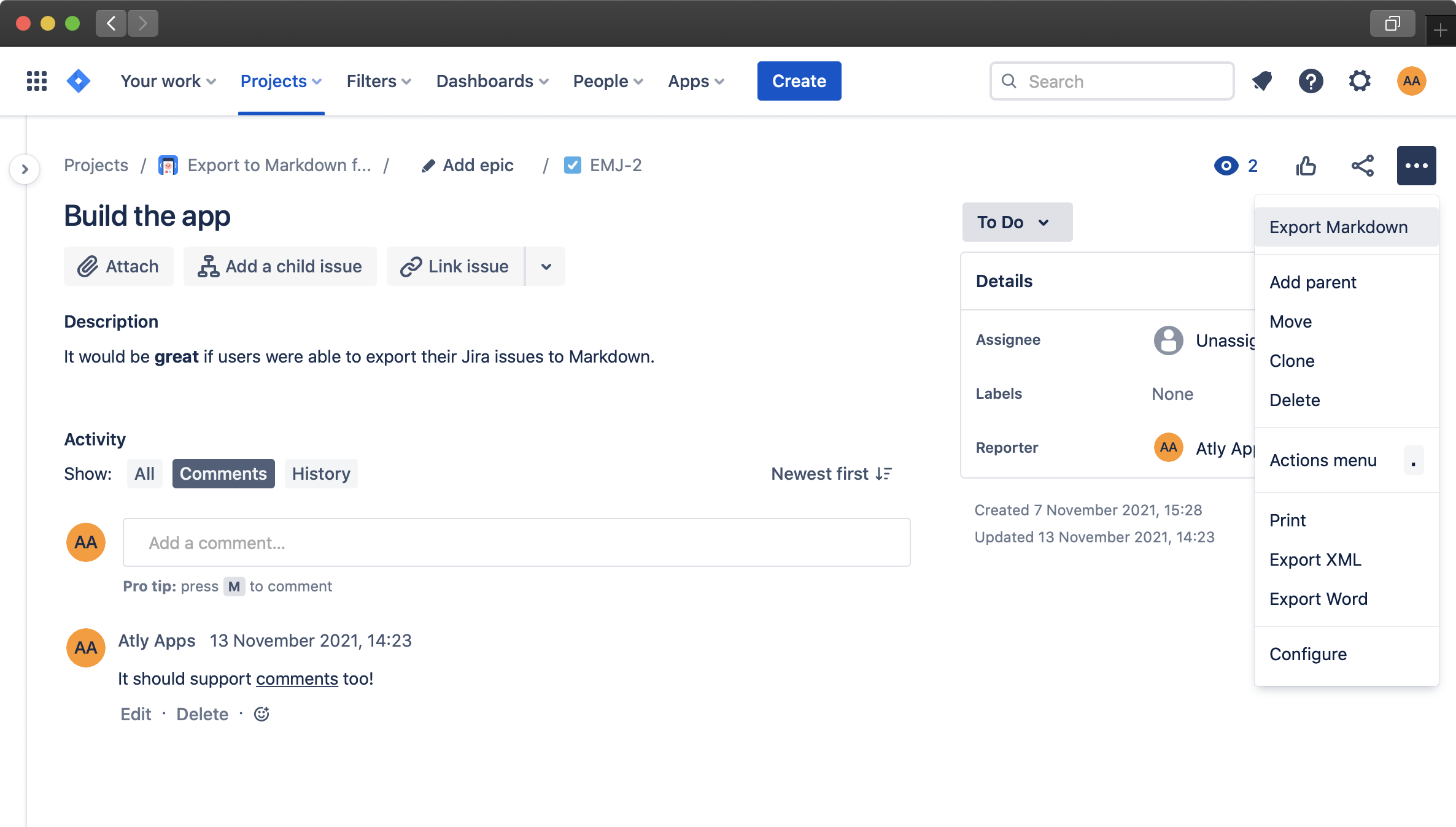In this screenshot of a website, the upper left corner features three circular buttons colored red, yellow, and green. Directly beneath these buttons, there is a white menu bar displaying several text options: "Your Work," "Projects," "Filters," "Dashboards," "People," "Apps," followed by a blue action button labeled "Create". To the right of this menu bar, there is a white search box.

Continuing below, the main content area begins with a secondary horizontal menu listing "Projects," "Export to Markdown," and "Add Epic" with a pencil icon. Adjacent to these options, there is a blue box with a white checkmark icon labeled "EMJ-2".

Further down, in bold black text, it reads "Build the App". Underneath this heading, there are three buttons: "Attach," "Add a Child Issue," and "Link Issue," which includes a pull-down arrow. Below these buttons, a section titled "Description" contains the text: "It would be great if users were able to export their JIRA issues to Markdown."

The "Activity" section follows, containing a sub-menu with the options "Show," "All," and "Comments" highlighted by a black button, and "History." On the right side of this sub-menu, the text "Newest First" is displayed.